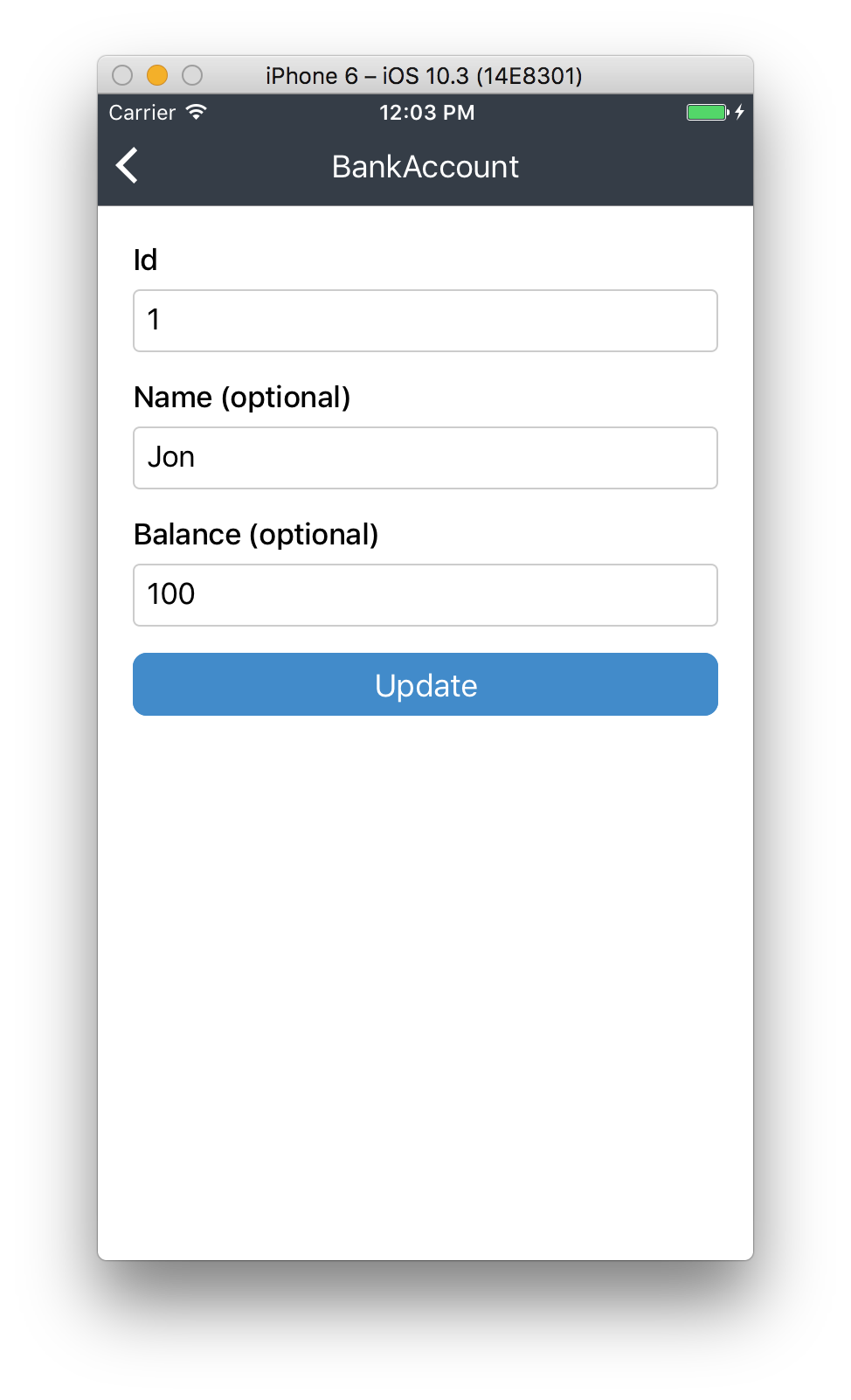The image is a screenshot of a financial app interface, specifically resembling a bank account summary, displayed in a landscape rectangular format. The screenshot features a clean white border and background. 

At its core, a shadow-enhanced floating rectangle is prominently centered. This central rectangle also extends longer horizontally than vertically. At the top of this rectangle, there is a light gray banner running from edge to edge. Within this banner, three circles are aligned to the left side. Centered within the banner, bold black text states "iPhone 6 - iOS 10.3 (14E8301)."

Directly underneath this banner, a gray bar extends horizontally across the width of the rectangle. The top left corner of this bar displays the label "Carrier." Positioned centrally within the bar, the current time reads "12:03 PM." To the top right of this bar, a fully charged battery icon with a green bar and an accompanying white lightning bolt is shown.

The bulk of the space below this gray bar is predominantly white, marked by three distinct text boxes. Centrally below everything, the words “Bank Account” appear in clean white text, subtly underscored to catch the viewer’s attention.

Overall, the layout is meticulously organized to ensure ease of reading and navigation, creating a user-friendly interface for financial management.